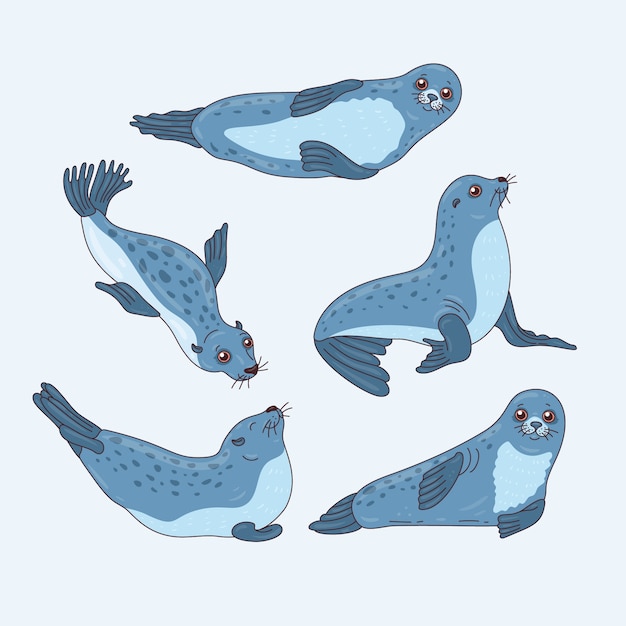The image is a rectangular cartoon drawing that is slightly taller than it is wide, featuring five seals against a very light bluish-gray background. The seals are depicted in shades of medium bluish-gray with lighter blue underbellies and grayer-blue fins. Each seal is in a distinct pose, contributing to a playful and dynamic scene. The first seal is lying on its side, gazing at the viewer with gentle brown eyes and a relaxed expression, flippers resting on its belly. The second seal, sitting upright in a backward L-shape, has one flipper tucked behind and appears to be staring off into the distance with a serene look. The third seal is in a side pose with closed eyes, flippers tucked underneath, and a peaceful smile. The fourth seal is diving headfirst, its wide eyes open in a curious expression, and flippers gathered at the back. The fifth and final seal is depicted as if swimming downwards, adding a sense of movement to the serene, underwater-themed illustration.